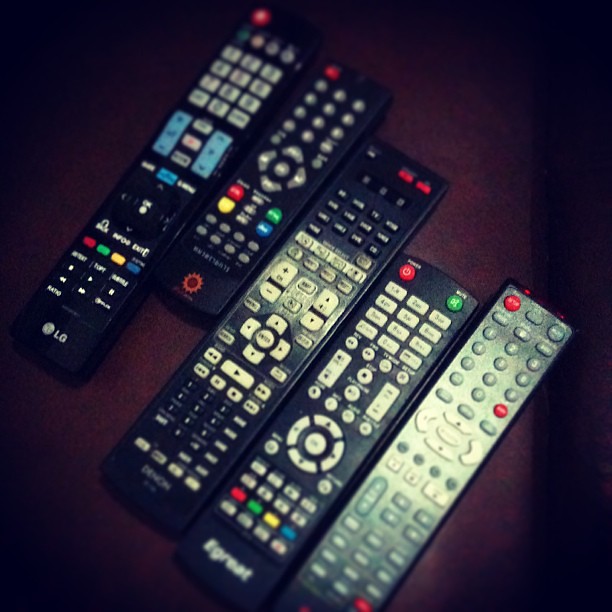In a dimly lit room, a photograph captures five distinct TV remotes arranged side-by-side at a 45-degree angle on a dark brown table or shelf, which fades into the surrounding darkness. Each remote is encased in black plastic, except for one with a silver face and gray buttons. The remotes are of various brands and feature an assortment of buttons in white, gray, and occasionally red, green, blue, and yellow. All remotes prominently display the traditional D-pad in their center, with most also having a red power button. The remotes vary slightly in size: four are roughly the same length, while the second remote from the left is about three-quarters the length of the others, featuring a mix of gray, white, and colored buttons. One brand, LG, is clearly visible. The composition of the photograph emphasizes the differences and similarities in design and function among the remotes.